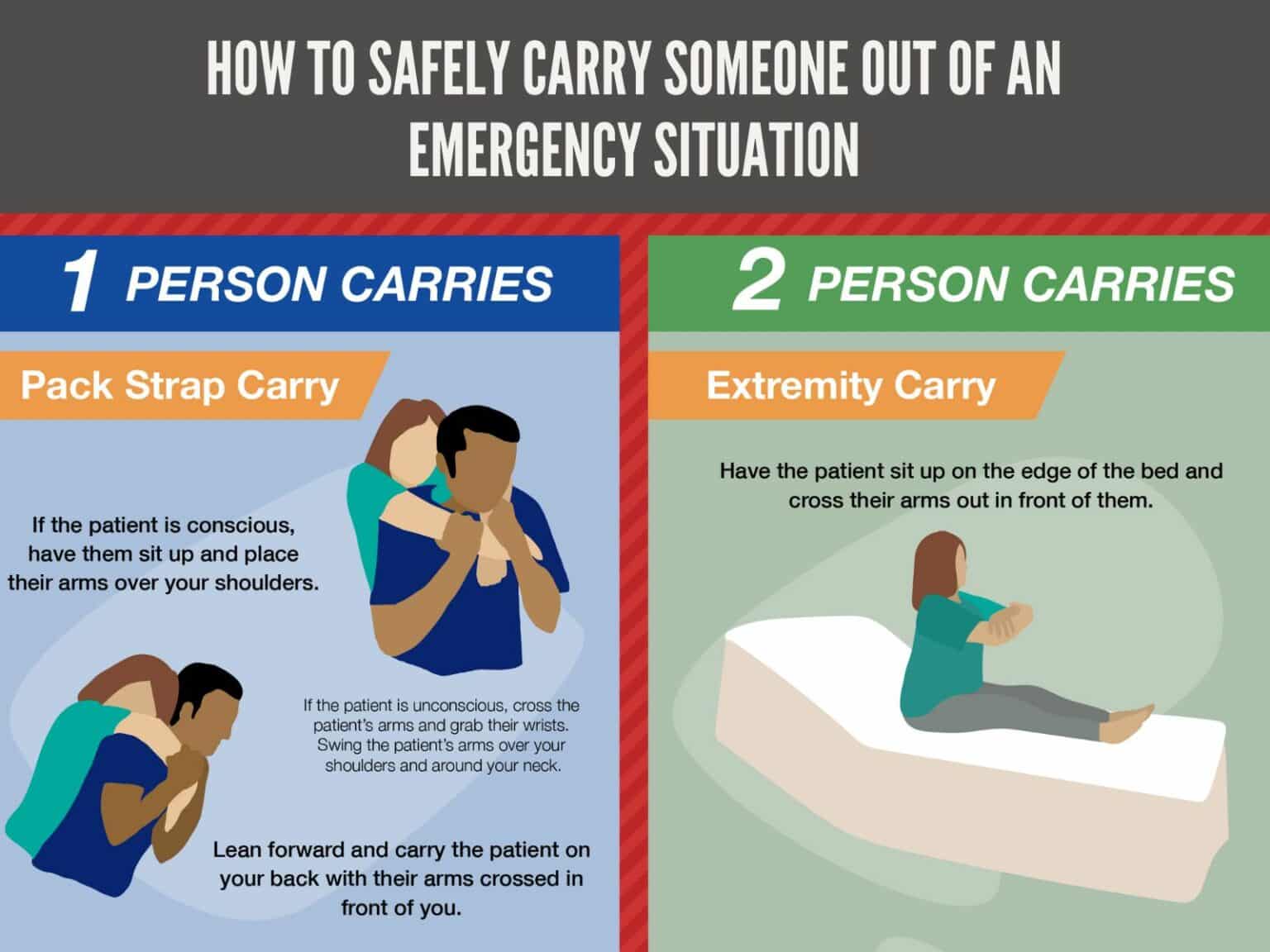The image is a detailed instructional poster on how to safely carry someone out of an emergency situation, presented in a landscape orientation with color illustrations and text. Across the top, a gray horizontal rectangle contains white all-capital text reading, "HOW TO SAFELY CARRY SOMEONE OUT OF AN EMERGENCY SITUATION." Below this, a red-orange section acts as a divider.

On the left half of the poster, a blue rectangle at the top contains the text "ONE PERSON CARRIES" in white. Below it, within a light blue background, are two illustrations demonstrating the 'Pack, Strap, Carry' method. The first illustration depicts a man carrying a woman over his shoulders from a rear view, and the second shows a side view of the same position with descriptive text in black surrounding the images.

On the right half, a green rectangle at the top holds the white text "TWO PERSON CARRIES." Below, a light green background shows an illustration labeled 'Extremity Carry.' This illustration portrays a woman seated on a white surface, facing right, with her arms folded over her chest. Additional explanatory text appears in black below the image. The poster combines instructional graphics with detailed text to provide clear and concise guidelines for emergency carrying techniques.